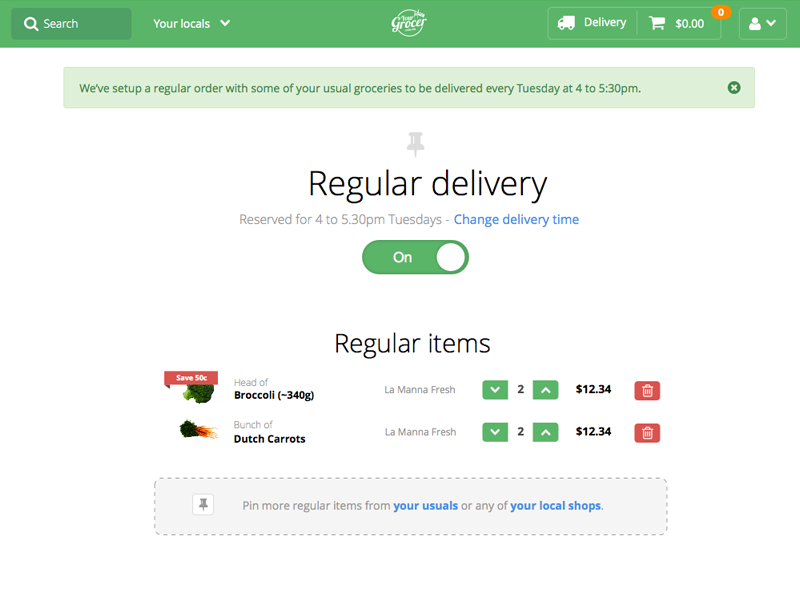Here's a cleaned-up and highly detailed caption for the image:

---

**Screenshot Description: Delivery Page Overview**

The screenshot displays a delivery page with several distinct sections and features. At the top, a green bar spans the width of the page. On the left of this bar is a dark green rectangular box labeled "Search," accompanied by a search icon. To the right of the search box is a dropdown menu labeled "Your Locals." Centrally located is the site or service name, partially obscured, but it includes the word "Grocer." To its right, there is a box with a van icon labeled "Delivery," followed by another box labeled "Cart," which shows the amount $0.00. Above the cart, a small orange circle displays the number zero. The farthest right feature in the top bar is a box with a person icon and a dropdown menu.

Below this top bar, a gray notification bar features green text stating, "We've set up a regular order with some of your usual groceries to be delivered every Tuesday from 4:00 to 5:30 p.m." There is a green circle containing an 'X' on the right side of this notification.

Beneath the notification bar, a pinned note symbol indicates a "Regular Delivery" section in black text. It notes that the slot is reserved for 4:00 to 5:30 p.m. on Tuesdays, with an option to "Change delivery time" in blue ink. An oval switch labeled "On" shows the white circle toggle to the right, indicating that delivery is active.

The content then lists "Regular Items." The first item displayed is a head of broccoli, parenthetically described as about 340 grams. An image of the broccoli is shown on the left, with a red banner indicating a “Save 50 cents” offer. To the right, the brand "La Manna Fresh" is specified. A green box with a down arrow (caret) and another with an up arrow allow quantity adjustment, currently set to 2. The price of the broccoli is listed as $12.34, with a red trash can icon for deletion to the right.

Following the broccoli, the second item listed is a bunch of Dutch carrots, illustrated with a photo of carrots including their green tops. It also belongs to "La Manna Fresh," with similar quantity adjustment options (currently 2) and a price of $12.34, along with a red trash can icon for removal.

The bottom part of the screenshot includes a gray dotted line around a light gray box, underlined by a pinned note symbol. The text within this box suggests adding more regular items from "Your Usuals" or with the option to select "Your Local Shops," both in blue ink for clickable links.

---

This caption provides a comprehensive description of the elements and layout within the screenshot, making it easier for someone to visualize the content without seeing the image.